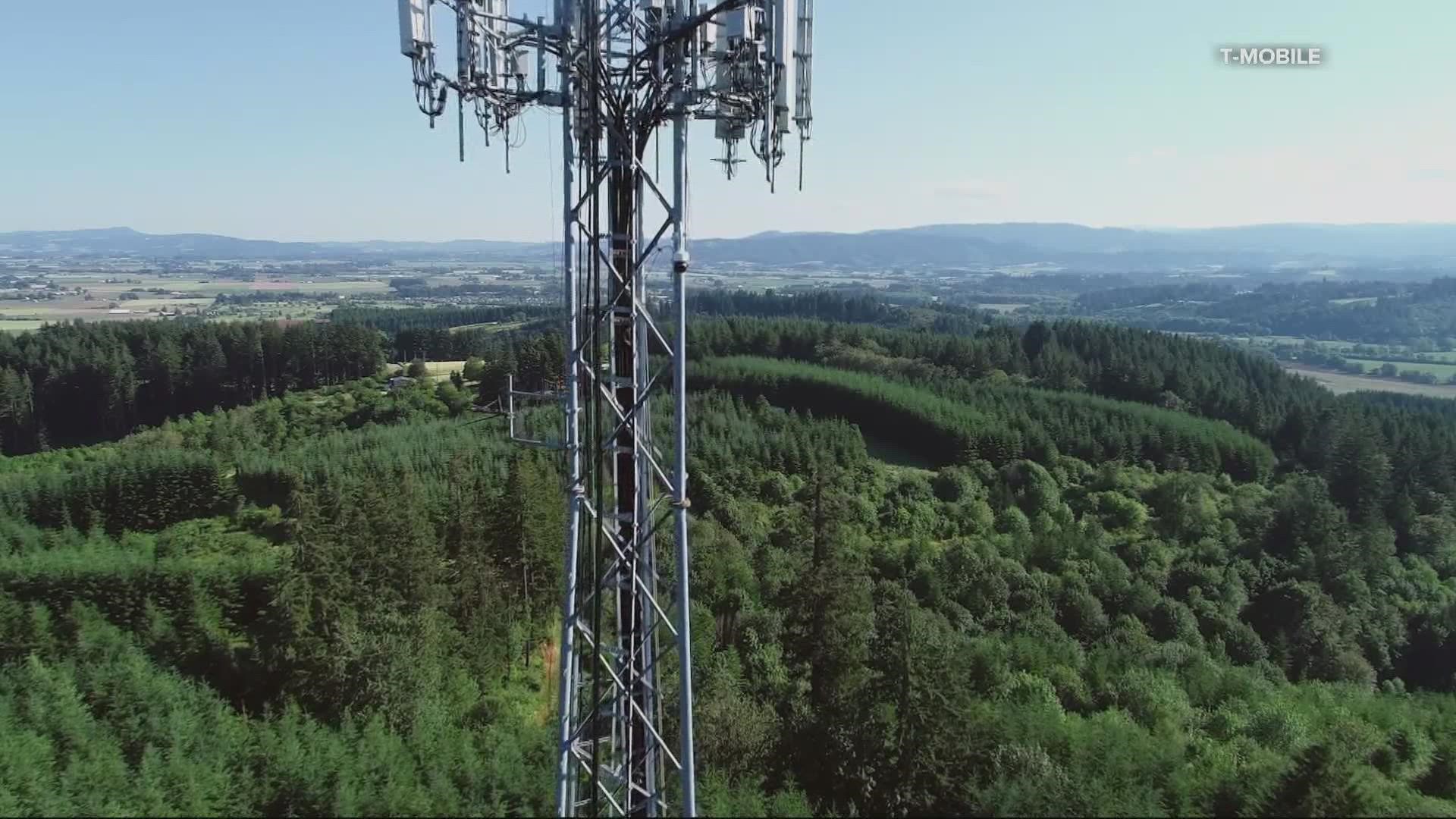The image features a prominent cell phone tower, identifiable by its towering steel structure and the various signal receptors attached near its top. The photograph is taken from a high vantage point, giving a sweeping view of the surrounding landscape. Rich greenery dominates the scene, with rolling hills and dense forests stretching out to the horizon. Mountains are faintly visible in the background under a clear, bright sky. The foreground showcases patches of cleared land interspersed among the trees, with small signs of civilization such as houses and vehicles in the distance. Notably, the top-right corner of the image is overlaid with the T-Mobile logo in clear, white text, suggesting the image may be part of a T-Mobile advertisement or infographic.